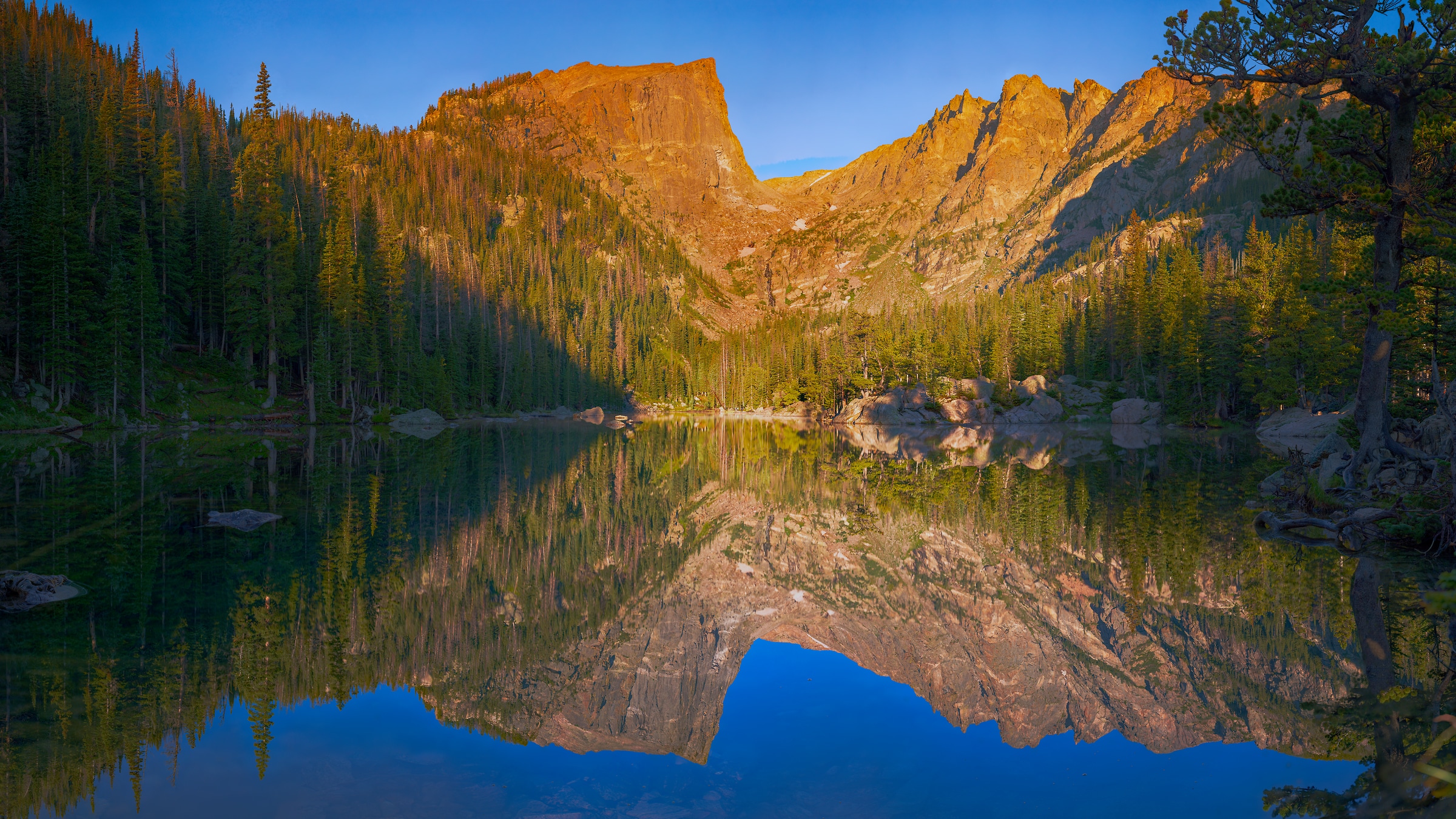This is a highly professional, full-color photograph capturing an outdoor landscape during a serene, clear sunrise. The horizontally rectangular image, devoid of any text or borders, showcases a completely still and reflective body of water, likely a lake or pond, mirroring the surrounding natural elements with exceptional clarity. The calm, blue water reflects the steep, reddish-brown and copper mountains that rise behind it, their sheer cliffs and rocky faces standing tall without any vegetative cover.

In the foreground, numerous stones and rocks dot the shoreline, adding texture to the tranquil scene. A striking row of skinny, tall pine trees, vibrant green with brown trunks, lines the center of the image vertically. Among them, a solitary tree stands out on the far right. 

The middle ground reveals more of the rugged shoreline and the dense forest, contributing to the depth of the photograph. Above, the sky boasts a bright blue hue without a single cloud, enhancing the overall clarity and peacefulness of the scene. The sunlight, illuminating the mountains with a warm, orange glow, adds a striking contrast to the image, emphasizing the natural beauty of this untouched, lifeless panorama.